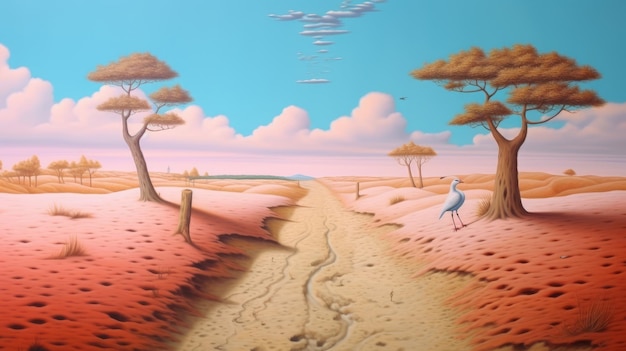The image is a surreal, fantasy scene that appears to be either a painting or a computer-generated piece with a smooth, soft art style. The landscape features vivid, reddish-pink soil and a sandy or biscuit-colored path that runs through the middle, resembling a dry riverbed. The sky is a bright, turquoise blue with a mixture of swirled, stylized clouds and more conventional puffy white clouds scattered throughout. 

On the right side, there are mature, brown trees with bushy leaves, standing out against the pink ground. A couple of tree stumps are also visible near these trees. In the foreground, there are additional brown trees and more in the background, contributing to the sense of depth in the artwork. A delicate, tall white bird with spindly legs, possibly a pheasant, is seen standing on the ground near the tree, adding a touch of life to the otherwise serene and dreamlike landscape.

This imaginative and peaceful scene is devoid of any human presence, and there are a few small, indistinct birds in the sky, enhancing the ethereal quality of the picture.